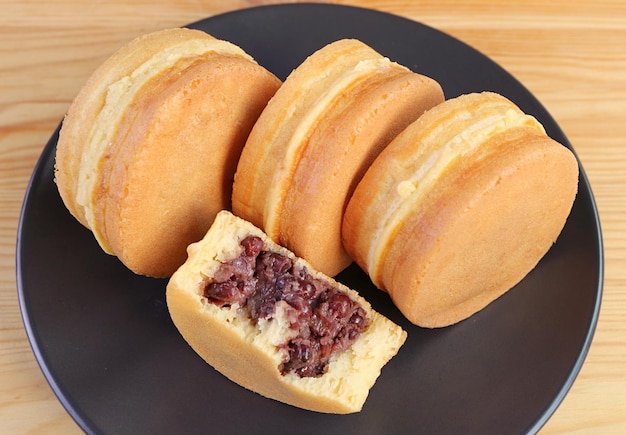Displayed in this photograph is a close-up of a black ceramic plate adorned with a subtle blue ring along its edge, all set against a light tan wooden table. Atop the plate, there are four Doriaki, beautifully arranged. Three of these golden-brown, cylindrical cakes are positioned on their sides, showcasing a lighter ridge encircling their middle. The fourth Doriaki is strategically cut in half, presenting a delectable cross-section with its filling side up. This cut half reveals a light yellow sponge cake enveloping a generous portion of thick, red bean paste filling that is slightly oozing out, offering a visual treat of its rich, creamy texture interspersed with discernible bits of beans. The slightly grilled tops of these pastries accentuate their inviting, fluffy appearance, making the entire setup a mouth-watering display of traditional Japanese confectionery.